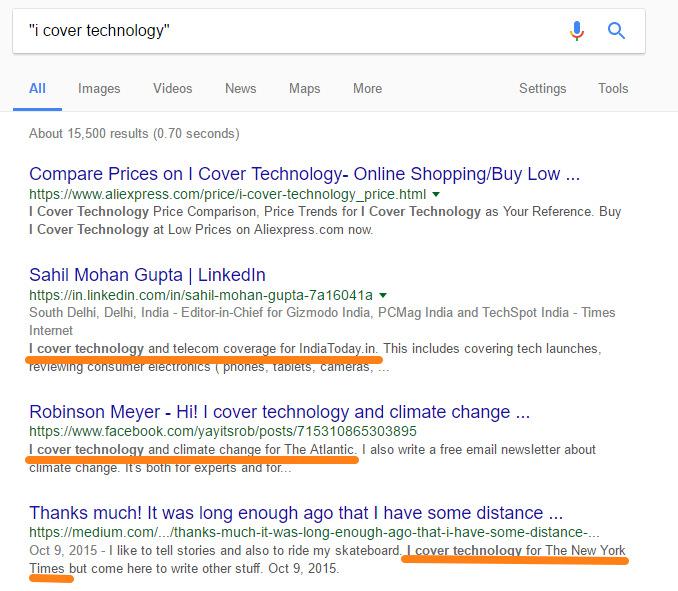The image displays a detailed search result page for "iCover technology." At the top, various options such as images, videos, news, maps, settings, and tools are available. The search query yields approximately 15,500 results in 0.70 seconds. Prominent search results include a price comparison for iCover technology on AliExpress, specifically at www.aliexpress.com/price/iCover_technology_price.html, emphasizing low prices and online buying options.

Further down, important individuals and their professional links are noted. Sahil Mohan Gupta, based in South Delhi, India, appears linked through linkedin.com/in/SahilMohanGupta7A16041A. He holds positions such as Editor-in-Chief for Govisno India, PCMag India, Techspot India, and is connected to Times Internet. His work involves covering technology and telecom in India, including tech launches and reviewing consumer electronics like phones, tablets, and cameras.

Also highlighted is Robinson Meyer, who focuses on covering iCover technology and climate change for The Atlantic. He mentions authoring a free email newsletter about climate change aimed at both experts and the general public. The text refers to a post dated October 9th, 2015, where Meyer mentions his interests in storytelling and skateboarding, as well as his association with The New York Times for topics other than technology.

A Facebook post from Robinson Meyer (facebook.com/yayitsrob/posts/715310865303895) reiterates his engagement with iCover technology and climate change for The Atlantic, and similar engagements for India Today.

The search results are visually emphasized with certain text portions underlined in gold.